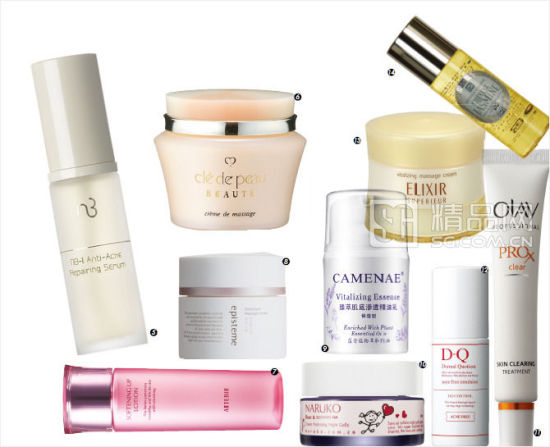This image features an array of skincare products displayed neatly. On the far left, there's a product with attractive packaging labeled "Anti-Acne Repairing Serum." It has a sleek plastic cap and the serum inside appears to be a white color. Next to the serum, there's a pale peach-colored jar branded with "DD Beauty." Below this jar, there is another jar, though the image is somewhat blurry, making the text on the jar difficult to read. Additionally, there is another jar which stands out due to its label with foreign writing, likely Chinese characters. This jar features the word "Kamine" and displays a graphic image of lavender, adding an aesthetic touch to the overall presentation. The combination of different shapes, colors, and text styles creates a visually engaging arrangement of skincare items.